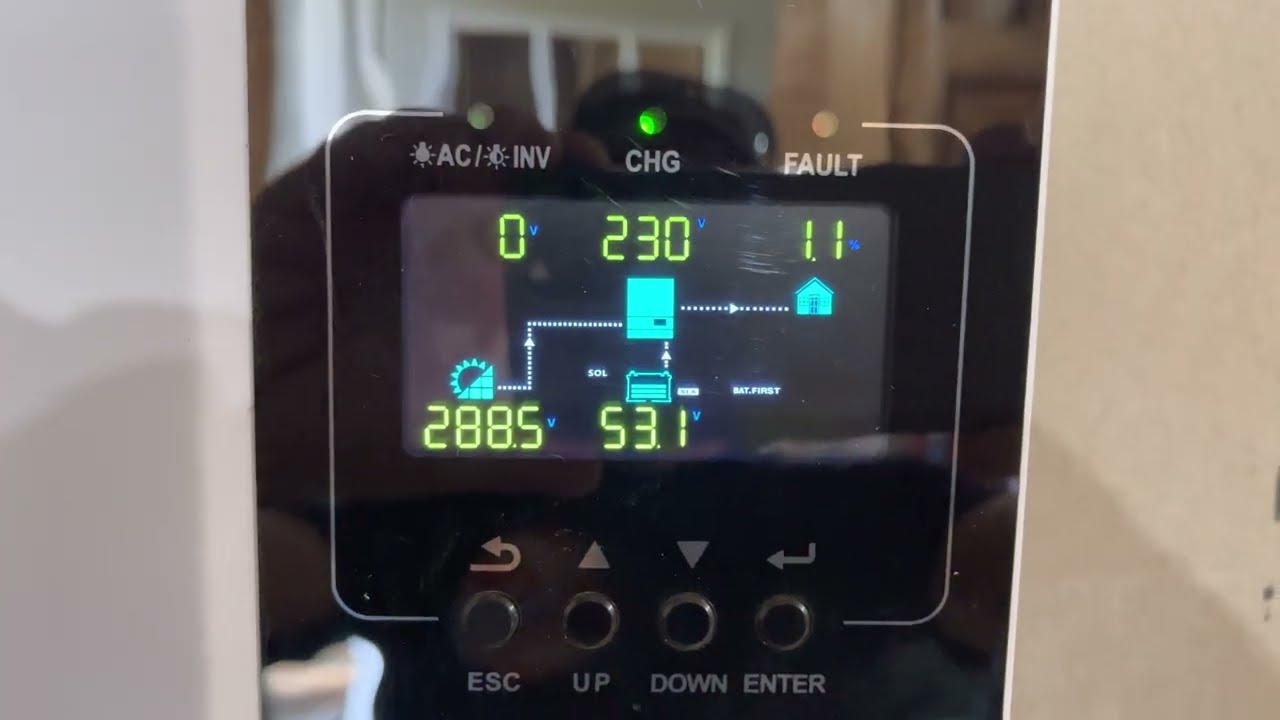The image depicts a close-up view of an electrical system monitor used to manage energy from solar panels and a battery. The screen on the monitor displays various measurements and icons. At the top, it shows readings like "0V", "230V", and "1.1%". Additionally, at the bottom, there are displays with "288.5V" and "53.1V". The monitor also displays acronyms such as "AC/INV", "CHG" with a green light indicating it's active, and "FAULT". The control buttons below the screen are labeled "ESC", "UP", "DOWN", and "ENTER". The screen also features a diagram illustrating the flow of energy from solar panels and a battery into a system, which then supplies power to a house. The image is well-lit, showing the monitor clearly against a white wall, with a subtle reflection of the person taking the picture visible on the display.